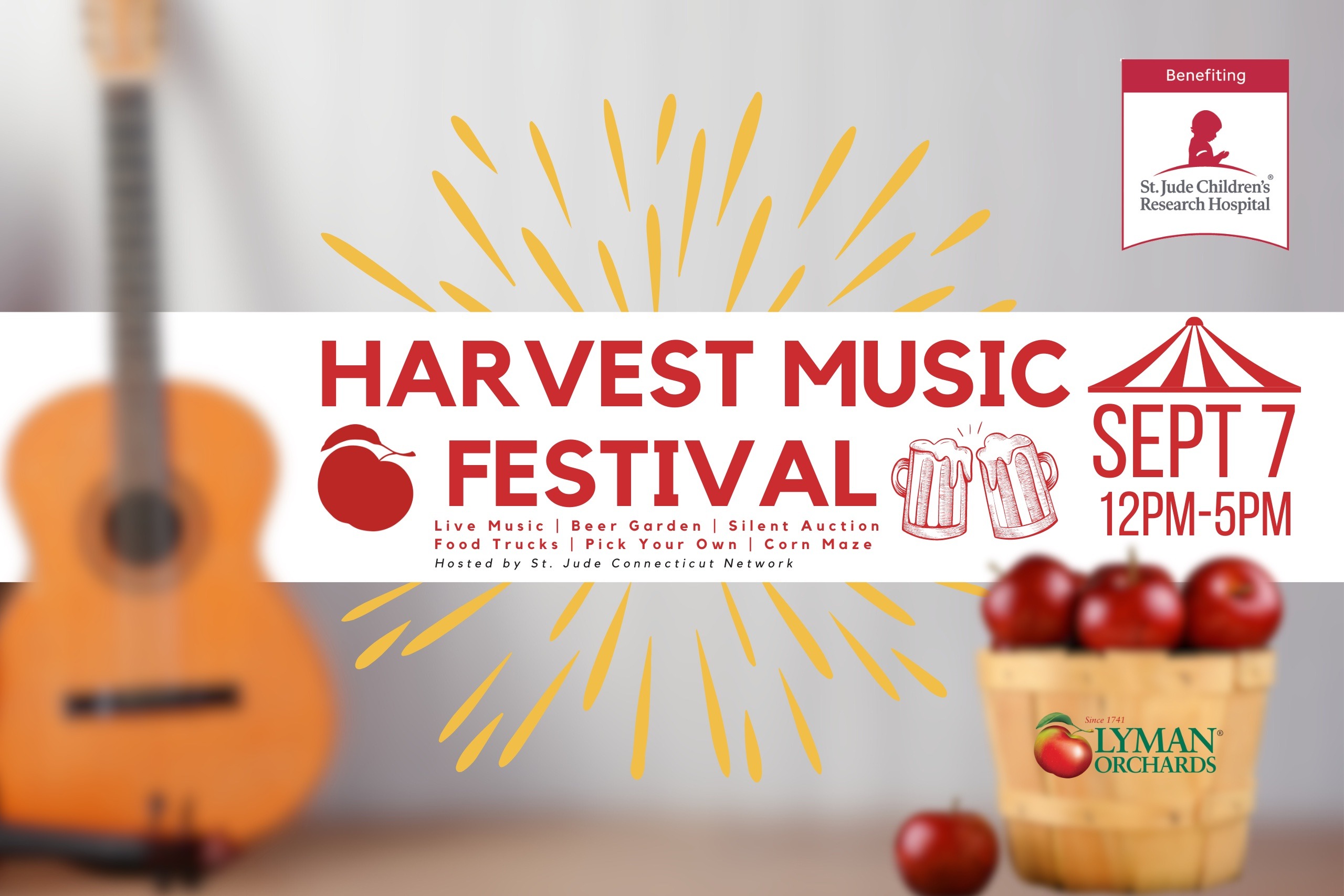The image is a horizontal, rectangular advertisement for an event with a gray background and a blurred brown flora-like image. On the right side, there’s an out-of-focus guitar leaning against the wall, while at the bottom right, there’s a basket labeled "Lyman Orchards," seemingly filled with apples. At the top of the poster, a small banner reads "Benefiting St. Jude's Children's Research Hospital." The central feature is a white banner with red writing stating "Harvest Music Festival" flanked by an apple and beer mugs. The event details, "September 7, 12 p.m. to 5 p.m.," are displayed next to this. Below the main banner are further red text details: "Live Music, Beer Garden, Silent Auction, Food Trucks, Pick Your Own, Corn Maze." In smaller, darker letters, it mentions that the festival is hosted by the "St. Jude Connecticut Network", reinforcing the philanthropic cause supported by the event.